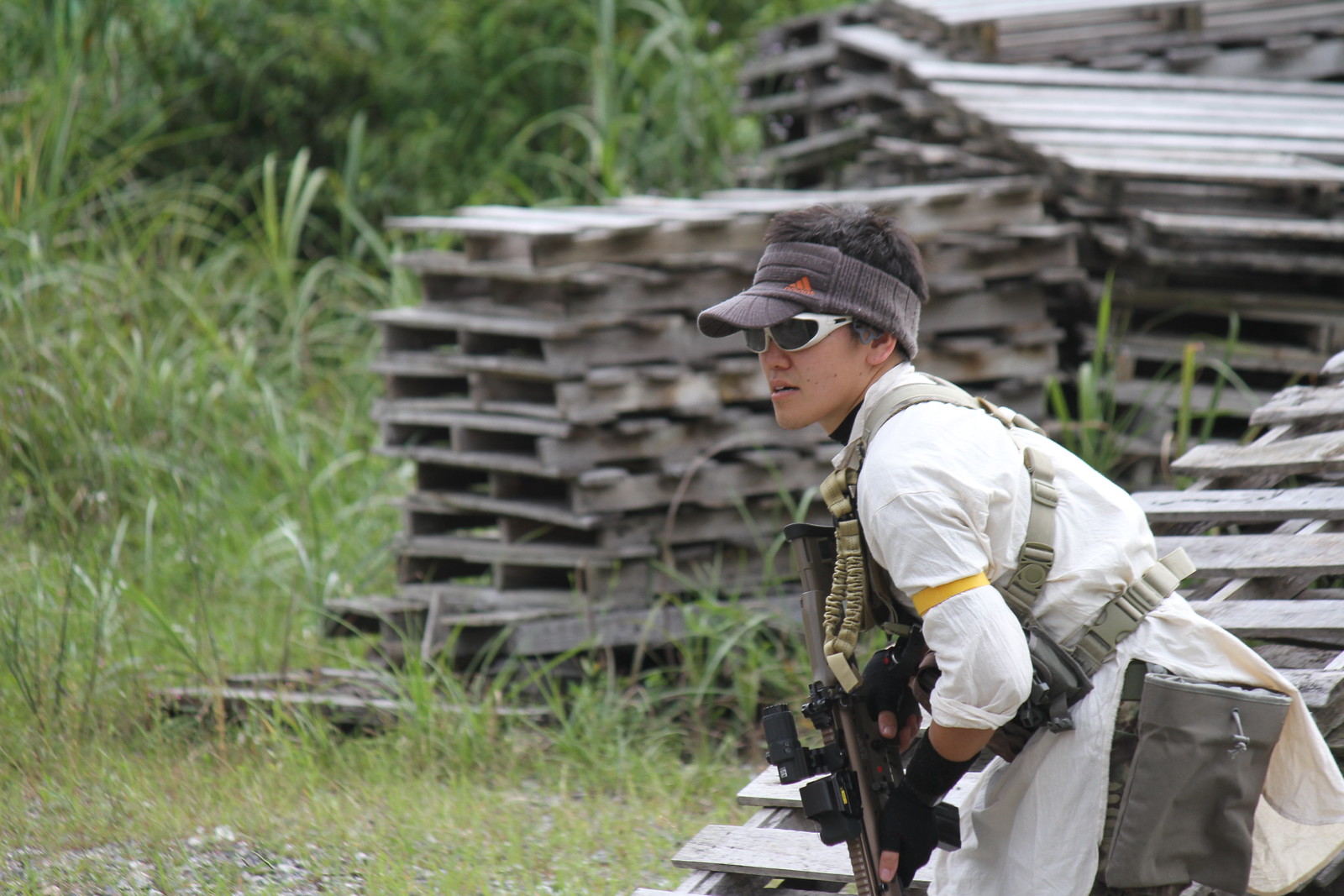In the image, an outdoor scene depicts a military exercise taking place in a grassy field bordered by a dense tree line in the background. Amidst this setting, numerous stacks of wooden pallets are scattered irregularly, with some piles positioned in the upper right, center, and directly behind the figure in the lower right-hand corner. The field itself features patches of gravel and rocks, particularly visible in the lower left-hand corner, interspersed with thin grass and taller plants.

A man, crouched and positioned in the bottom right corner of the image, commands immediate attention. Wearing military gear, he is equipped with a white long-sleeve shirt, brown pouch, gray baseball-type hat, and white sunglasses. The man, who has short brown hair and olive skin, holds a gun downwards in his arms. The overall scene is bathed in daylight, with the composition balancing the detailed greenery and the structured chaos of the wooden pallets, giving a stark contrast to the orderly military presence. There is no text in the image to distract from its vivid details and realistic setting.